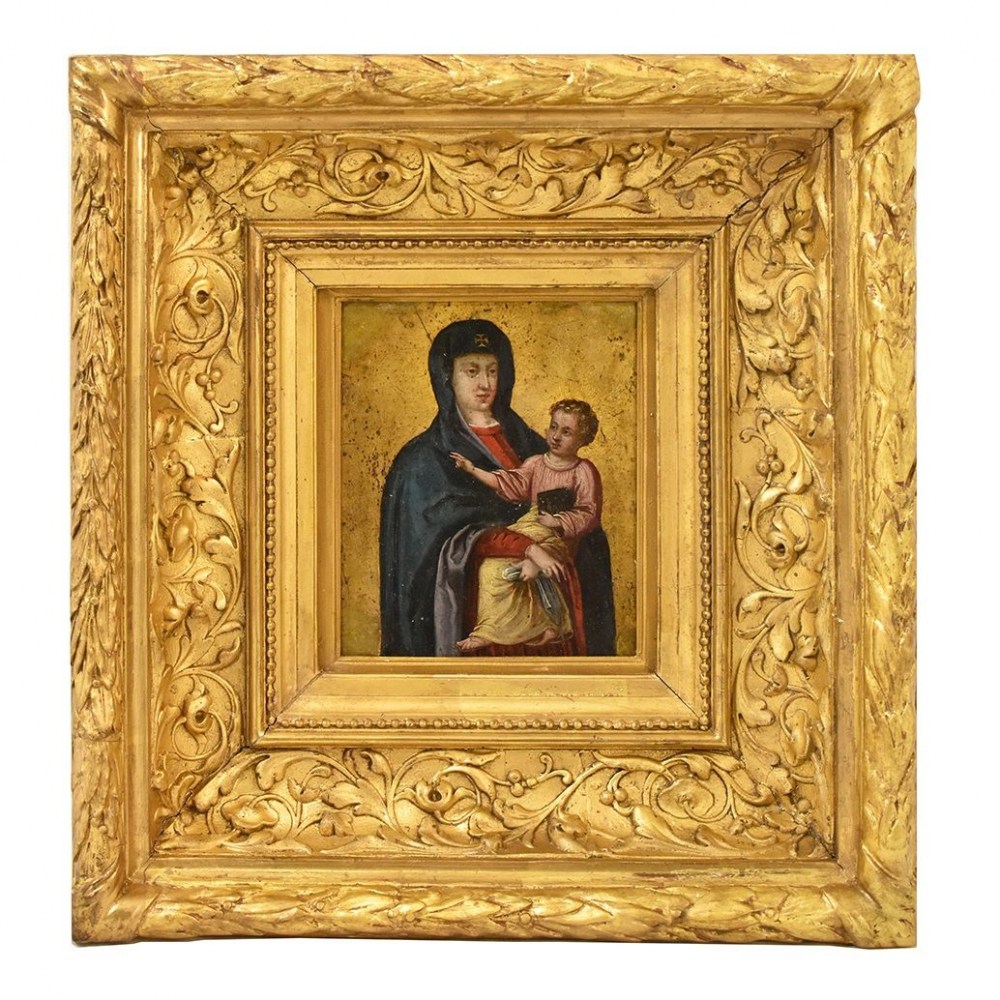This is a full color, square photograph of a staged, indoor scene illuminated by artificial light. The image prominently features an ornately designed gilded frame with seven distinct borders, each varying in complexity from simple polished wood to intricately carved floral and leaf patterns. The outermost layers of the frame showcase finely detailed carvings of flowers, leaves, and berries, all rendered in gold. Moving inward, the layers transition through various gold textures, from rectangular borders with a dotted pattern to delicate designs, culminating in the central portion.

Inside the luxurious frame is a very old-looking painting that mirrors the golden tones of its enclosure. The centerpiece of the painting depicts a solemn scene of a mother and child, likely representing Mary and Jesus, given their attire and demeanor. The mother, attired in a dark blue cloak over a red dress, gazes downward with a serious expression. She cradles the child—who has blonde curls, bare feet, and a long robe that transitions from pink to yellow—tenderly around the knees. The child, who looks up at the mother, clutches what appears to be a small black book while a blanket is draped around the lower part of the body. This carefully composed image exudes a timeless, almost sacred quality, enhanced by the intricacy of the framing.